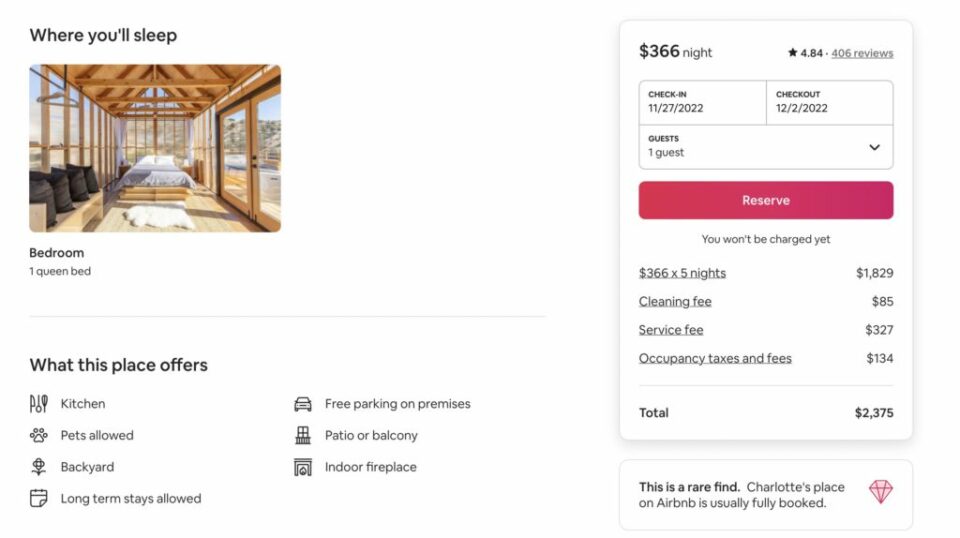The image showcases a detailed listing on a travel website, specifically for an Airbnb rental named "Charlotte's Place." In the upper left corner, the section titled "Where You'll Sleep" features an inviting photograph of a room with a bed. The room is exceptionally bright, filled with natural light streaming through numerous large windows. Below the image, it specifies "Bedroom - 1 Queen Bed." 

The amenities are listed in black text, including a fully equipped kitchen, pet allowance, a spacious backyard, and options for long-term stays. Additional features highlighted on the right side of the image include free parking on premises, a patio, a balcony, indoor fireplace, and the accommodation’s nightly rate of $366. 

Charlotte's Place boasts an impressive rating of 4.84 stars, based on 406 reviews. The booked dates visible are from November 27, 2022, to December 2, 2022, for one guest. A prominent pink "Reserve" button indicates that for these five nights, the subtotal is $1,829. Additional costs are broken down as follows: cleaning fees of $85, service fees of $327, and occupancy taxes and fees, culminating in a total of $2,375. 

A noteworthy point emphasized at the bottom of the listing is that "Charlotte's Place on Airbnb is usually fully booked," indicating its popularity and demand.